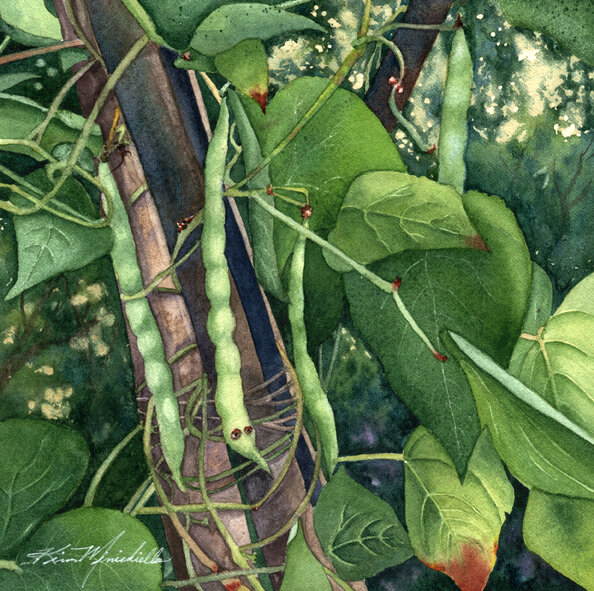This detailed artwork depicts a lush natural scene set in a forest, centering on a bean plant that is both vibrant and intricate. Most of the image is bathed in green hues, primarily featuring large leaves that are predominantly green with occasional reddish tips. Dominating the composition is a prominent tree running vertically through the middle, from which several pea pod-like beans hang down. There are at least four pods visible, with one in the center intriguingly illustrated with eyes on the bottom tip.

The artwork also showcases a sturdy, brown woody stem to the left, which serves as an anchor for the plant. Bean vines entwine around this supporting wood and extend throughout the drawing, contributing to the rich, verdant scenery. The background is filled with additional forest greenery and another faintly visible tree, enriching the sense of depth. The artist's initials, elegantly written in white cursive, can be found in the bottom left corner, subtly blending into the naturalistic setting.